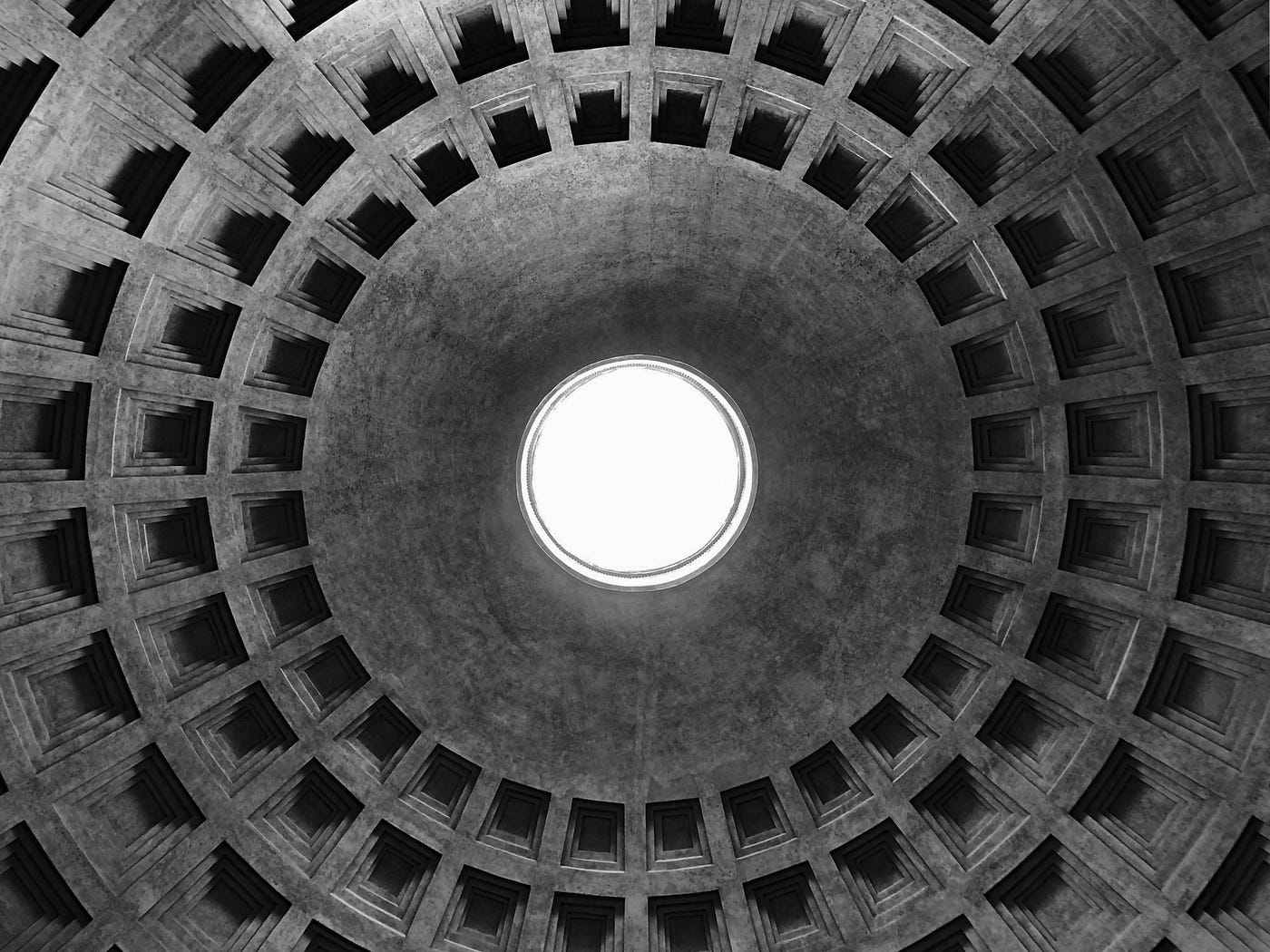The black and white horizontal rectangular image depicts an architectural interior, likely under a cupola of a historic building such as a chapel. Dominating the scene is a concentric circular design centered around a white, light-filled opening. Surrounding this central light, multiple concentric circles are fashioned from chiseled rectangular and square patterns in a radiating sequence. The immediate circle around the light is marked by a gray, molded material, potentially plastic or stone-like in texture. Each subsequent circle features increasingly larger squares, etched deeply to create a shadow effect that enhances the depth and intricacy of the design. The concentric squares within each larger square add further layers of detail. The combination of shapes and shadows crafts an ornate and visually compelling pattern on the ceiling.